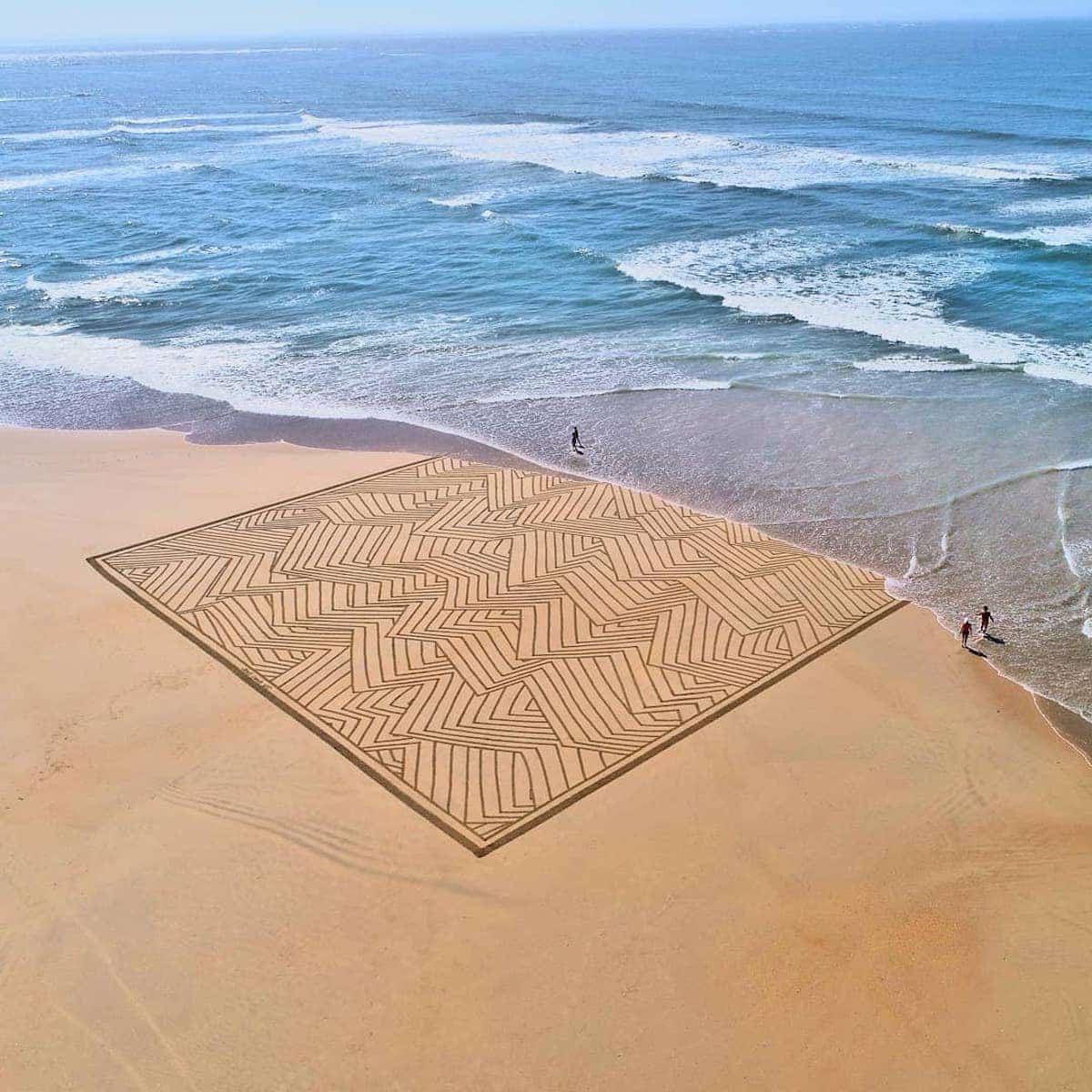The aerial photograph, likely taken by a drone, captures a serene beach scene showcasing both natural and artistic elements. The shoreline runs from the upper left, curving to the right, and descending sharply to the lower right. Gentle waves, distinguished by white surf, meet the sandy shore, transitioning into the deep blue ocean that stretches to the horizon, beneath a sliver of light blue sky. Dominating the scene in the center of the image is a large, intricate sand sculpture shaped into a geometric square. The design features numerous ridges and lines forming a detailed pattern reminiscent of an abstract painting. This sand art is bordered by more solid lines, creating a distinctive frame within the beach. As the tide recedes, parts of the sculpture have started to be gently washed away by the advancing waves, hinting at its ephemeral nature. There are three people depicted in the scene: two on the right side near the middle of the image and one near the center, possibly wearing a hat. Their presence adds a sense of scale and life to the tranquil, artistic setting.